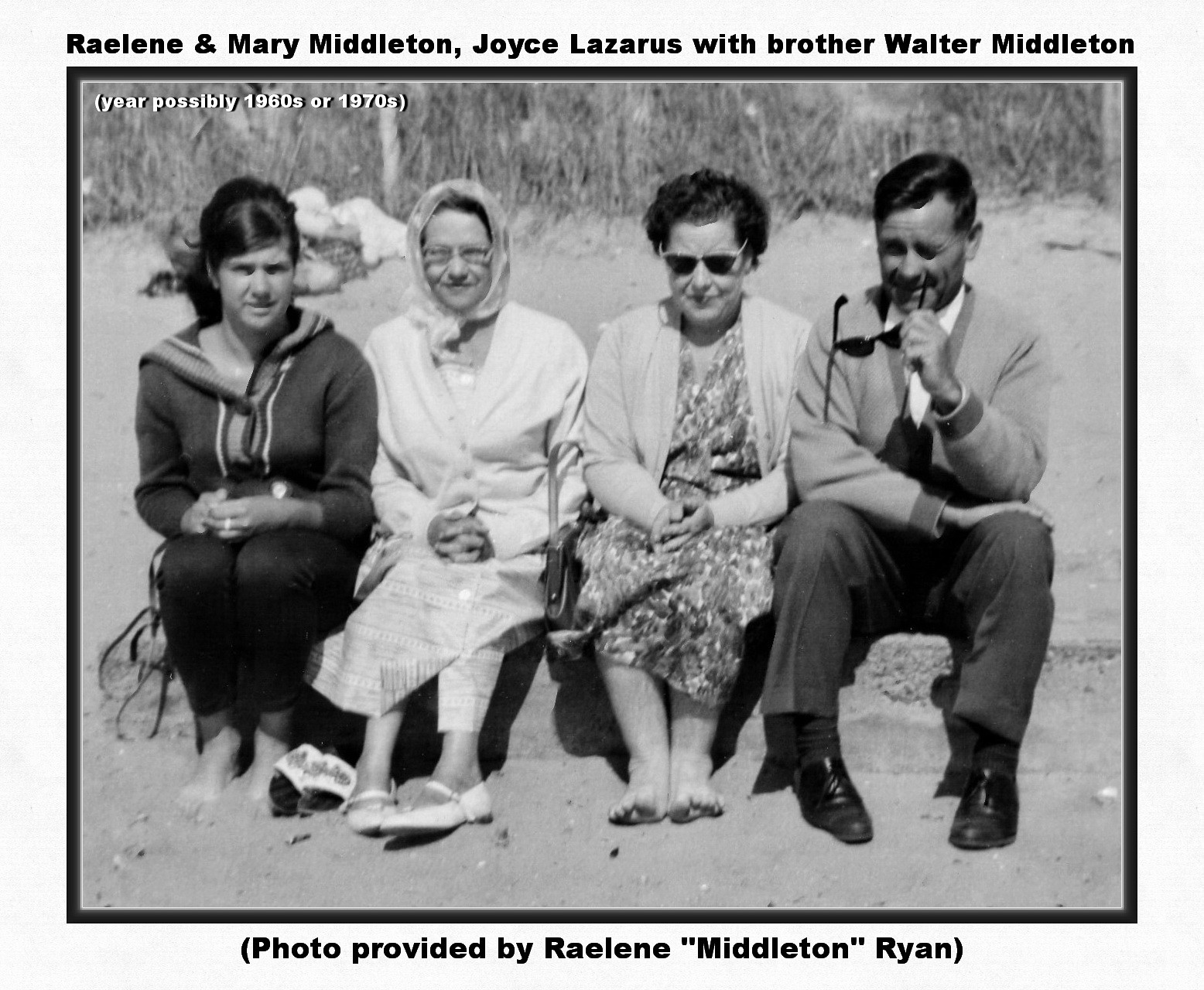This black-and-white photograph appears to be from the 1960s or 1970s, as indicated by white text in the upper left corner. It portrays four individuals seated on what seems to be a cement curb with sand and vegetation in the background, possibly on a beach. From left to right, the individuals are: 

1. **Raylene Middleton** - A younger woman dressed in black pants and a button-up sweater, who appears to be barefoot.
2. **Mary Middleton** - An older woman wearing a white dress with a scarf over her head.
3. **Joyce Lazarus** - An older woman dressed in a dress and a jacket, complete with sunglasses, who also seems to be barefoot.
4. **Walter Middleton** - A man attired in a V-neck sweater over a white shirt, black pants, and black dress shoes, holding sunglasses in his left hand.

At the top of the photo, black text identifies the individuals: "Raylene and Mary Middleton, Joyce Lazarus with brother Walter Middleton." Below the image, black text reads: "Photo provided by Raylene 'Middleton' Ryan."